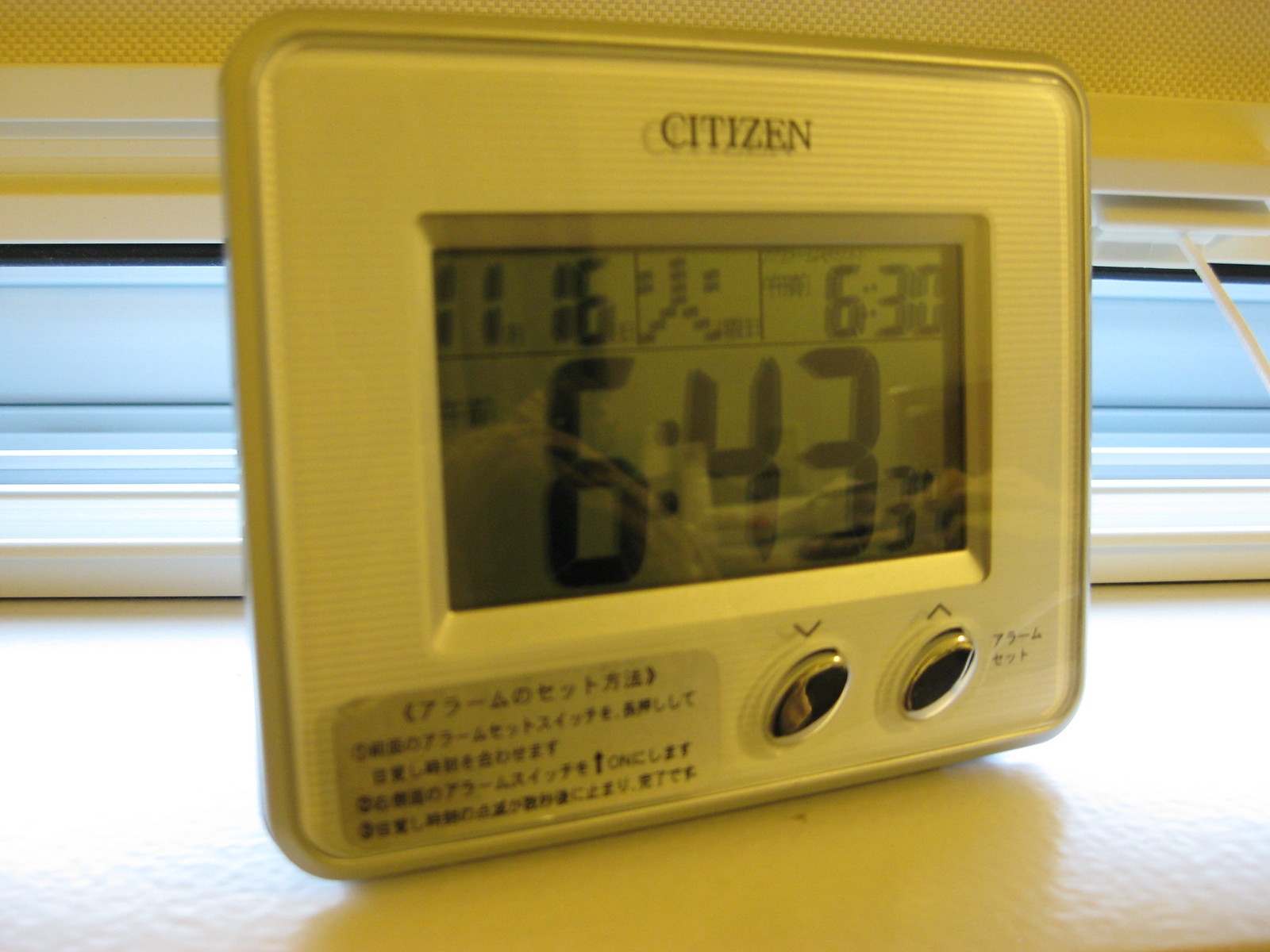This photograph features a small digital clock, predominantly white in color, with the brand name "Citizen" at the top. The clock’s face is comprised of several displays. The main display in the center shows the time as 6:43:34. Above this, there are three smaller horizontal displays: the leftmost reads 11:16, the middle contains an unidentifiable triangular shape, and the rightmost displays 6:30. At the bottom of the clock face, there are two silver, oval-shaped buttons. This clock is placed on a white windowsill, and appears to be backed by a window with the blinds drawn.